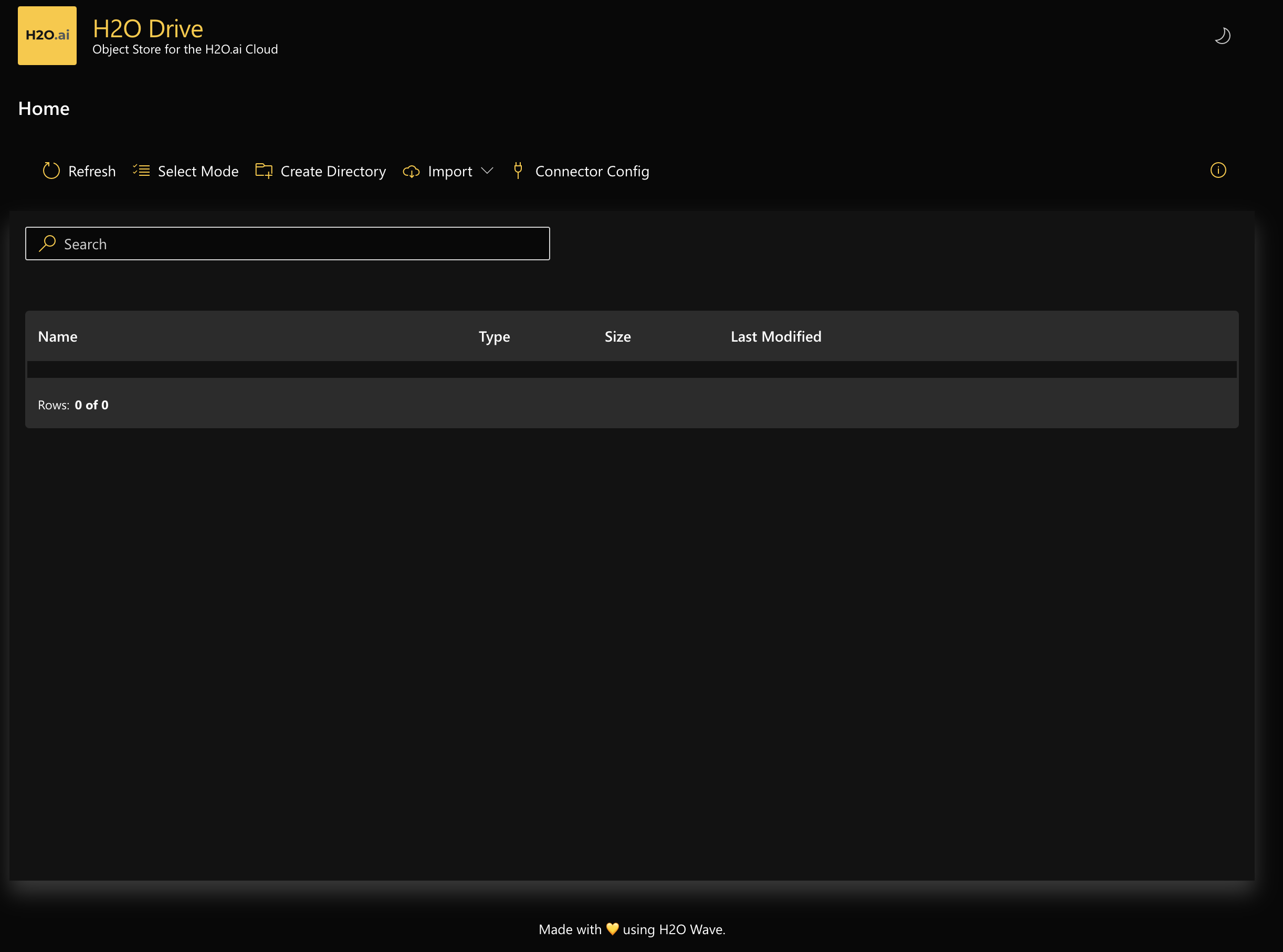At the top left-hand corner of the image, there's a yellow box labeled "h2o.ai," accompanied by text that reads "h2o drive, object store for the h2o AI Cloud." In the top right-hand corner, an icon of a moon is situated below which lies a navigation bar with options such as "Home," a refresh button, a "Select Mode" dropdown, "Create Dictionary," "Import," "Configure Connector," and a help icon resembling an "i." Adjacent to these controls is a search bar designed for user inquiries.

The main section of the interface appears to be a table format, structured with columns that are titled "Name," "Type," "Size," and "Last Modified." Currently, there are no entries in the table, as indicated by the "0 out of 0 rows" status. Finally, at the very bottom of the image, there is a footer that reads "Made with love using h2o Wave."